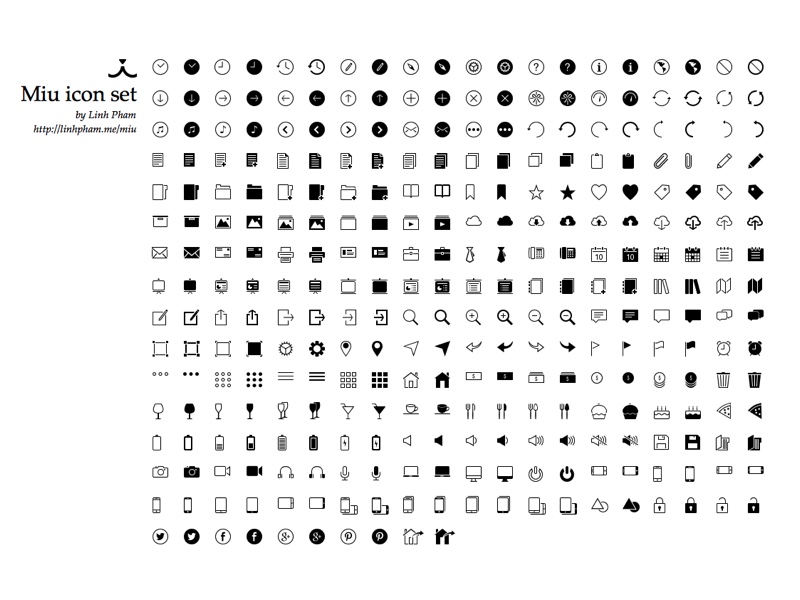This black-and-white image depicts the "MIU Icon Set" by Lin Pham, accessible at http://linpham.me/miu. The icons are arranged in a grid format, with 20 columns and 15 rows, except for the last row which contains 10 icons. The set features an extensive variety of computer-related symbols, including cursors, maps, stars, folders, and emojis. Additional diverse icons include hearts, paper airplanes, utensils, microphones, wine glasses, garbage pails, mobile phones, magnifying glasses, printer icons, martinis, birthday cakes, pizzas, headphones, cameras, houses, and different lock states. These symbols represent common UI elements and functions, suitable for various digital applications.